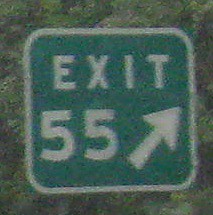This photograph prominently features a green highway exit sign with a square shape and noticeably rounded corners. Encircled by a white border, the sign displays the word "EXIT" in bold, white, sans-serif font. Directly beneath this, the number "55" is also presented in white, accompanied by an arrow pointing diagonally towards the top right, indicating a northeast direction. The background, although largely obscured by the sign itself, reveals a dense area of greenery, which appears to be a mix of trees and shrubbery, with varying shades of green and darker shadows. The image captures the exit sign in such close focus that it occupies almost the entire small square photograph. The overall fuzziness suggests that the image may have been either digitally zoomed in or is a photograph of another photograph.